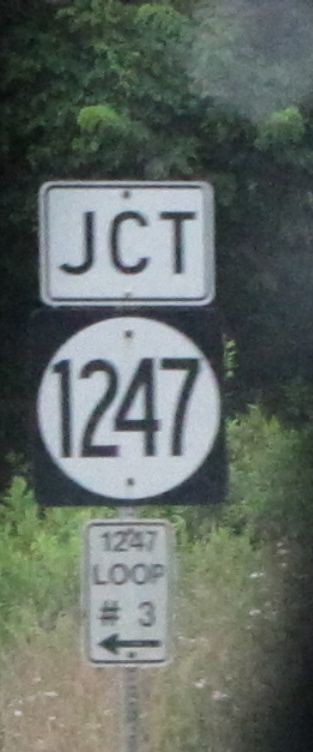The image is a vertical rectangle, thin and tall, appearing as a slightly grainy and blurry yet discernible photograph. It depicts a highway street sign set against a daylight outdoor background featuring tall green trees in the upper half and smaller, almost yellowish-green bushes and grasses in the lower half. Central to the image is a metal stainless steel pole supporting three stacked, vertical signs. The top sign is a white rectangle with black trim and text that reads "JCT". Below it, a square black sign with a white circle in the center displays the number "1247" in black text. The bottommost sign is a vertical rectangle, white with black trim, which reads "1247 Loop #3" in black letters accompanied by a left-pointing arrow. The entire scene suggests an older photograph, potentially sourced from Google Maps, and is tightly cropped to focus solely on the vertical alignment of the signs against the lush, wooded background.